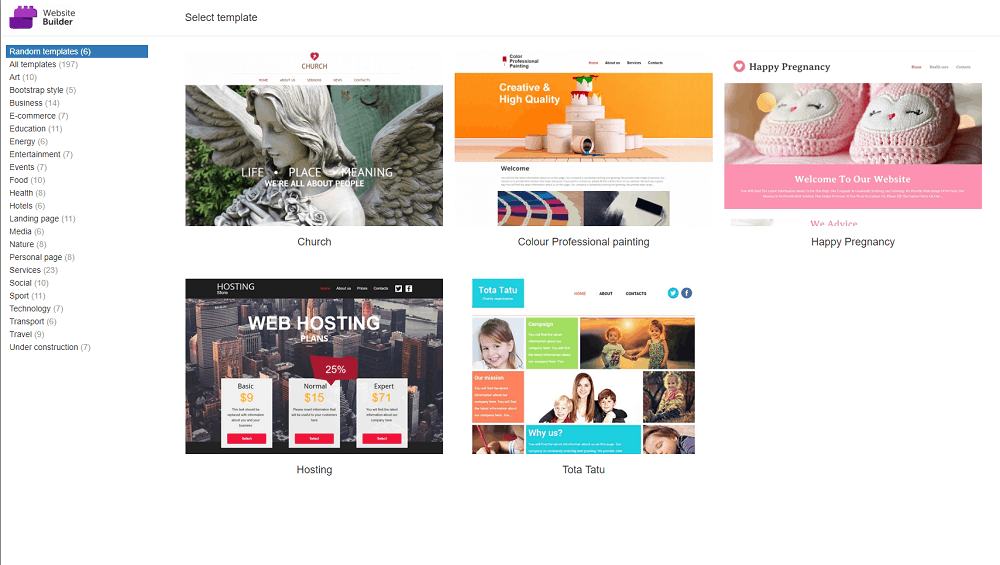This image features a screenshot from a web hosting service or website builder platform. In the upper left-hand corner, the platform is identified as "Website Builder," denoted by an icon of two purple blocks resembling Legos. At the very top of the interface, a prompt labeled "Select Template" invites users to choose from a variety of website templates. Down the left-hand side, a comprehensive list categorizes these templates, showcasing the number of options available in each category. Categories include: All Templates, Art, Bootstrap Style, Business, E-commerce, Education, Energy, Entertainment, Events, Food, Health, Hotels, Landing Page, Media, Nature, Personal Page, Services, Social, Sport, Technology, Transport, Travel, and Under Construction.

On the right side of the interface are previews of available templates. The first template preview is titled "Church" and features a mock-up with a statue of an angel alongside white text that reads "Life, Place, Meaning." The middle template is called "Colour Professional Painting," notable for the British spelling of "colour," indicating that the platform may be tailored for users in Commonwealth countries such as the UK, Canada, or Australia. It presents a visually appealing design aimed at the painting industry. Next, "Happy Pregnancy" displays a pair of adorable crocheted baby slippers. Below this, the "Web Hosting" template is characterized by a sleek and professional business-like design. Finally, the "Tota Tattoo" template provides a versatile layout ideal for showcasing photographs, allowing users to create collages and add text blocks, catering specifically to tattoo artists or studios.